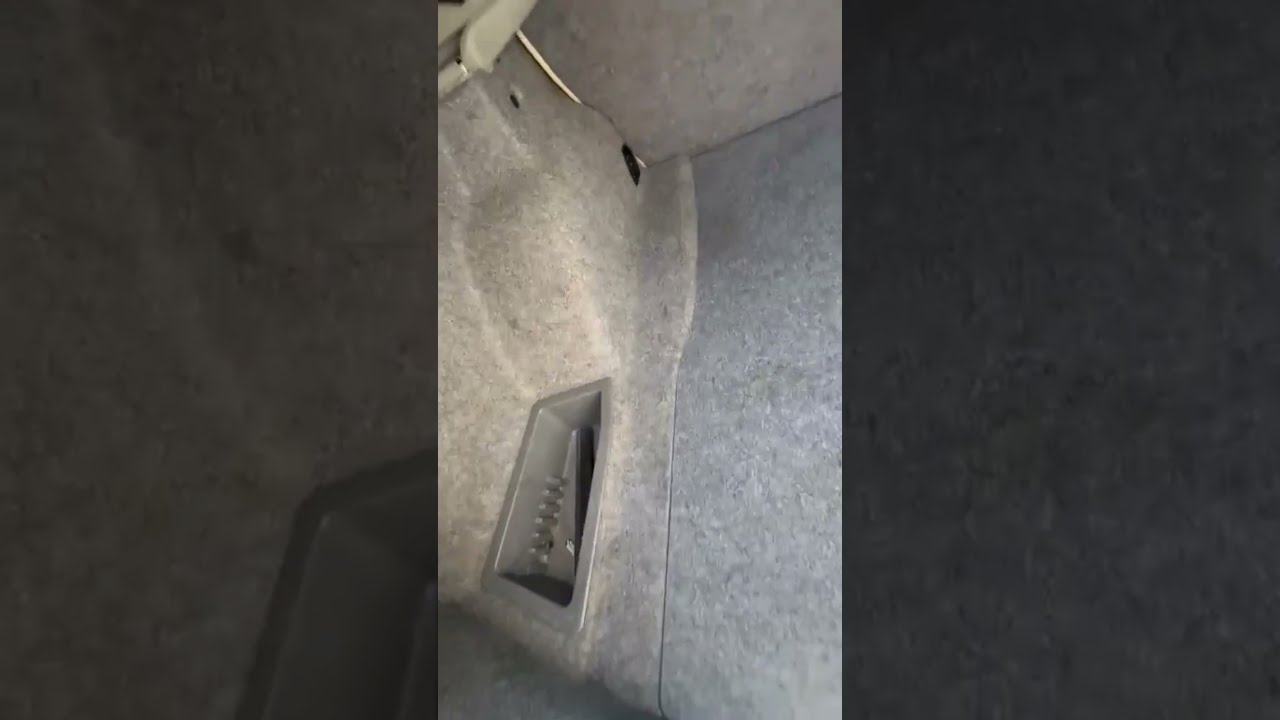The image depicts a close-up view inside a vehicle's trunk area, featuring a gray wall and floor as the background. On the left side of the image, a silver rectangular tray rests on a low platform, several inches above the ground. A beige plastic frame is situated on a higher platform at the top left corner, with a white wire extending from the tray down to the ground. The trunk or console area shows a cloth texture, indicating the inside finish of the vehicle. There is a small, brown rectangular cup-like area and a metal rod with a golden hue in one corner. In the distance, several holes and plastic parts are visible, contributing to the gray and brown flat texture of the trunk's interior. The console area also features a gray, deep empty container, with the adjacent seat interiors in shades of gray and light blue, set against a black background.